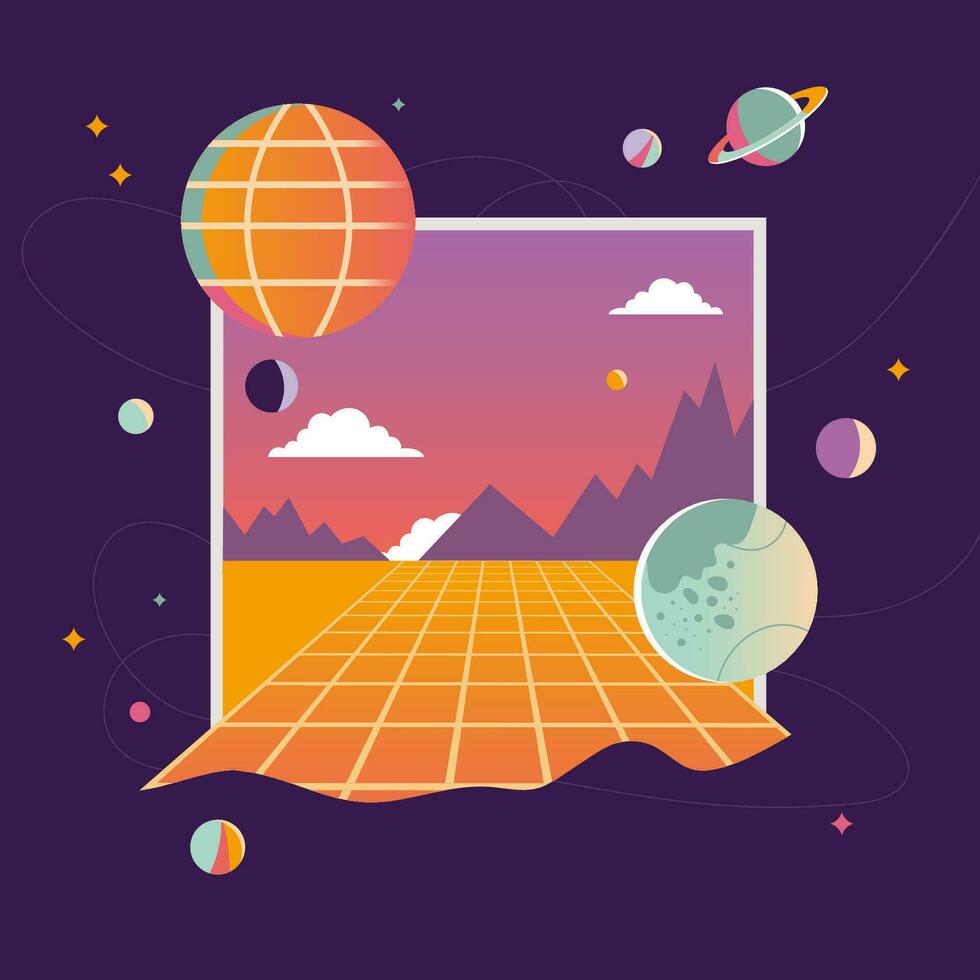This vibrant and futuristic image, featuring a deep purple background, is centered around a square illustration depicting a stylized, abstract nature scene. The central square, outlined in white, showcases a checkerboard-like ground that is predominantly orange, leading into simplistic, cartoonish mountains in the background. These mountains are depicted merely as line drawings without detailed features.

Above the mountains, the sky is a lighter shade of purple, dotted with three white clouds. Two celestial bodies, one resembling a yellow sun or moon with a white highlight and another larger purple ball with a greyish-white mark, float in this setting. Adding to the surreal nature of the scene is a grid that extends from the foreground to the base of the mountains, enhancing the geometric theme of the poster.

Encircling this central square are various space-themed elements, including stars, planets, and objects that mimic solar system bodies. Notably, there's an image of a planet with a ring, resembling Saturn, positioned in the upper right, alongside additional planets and stars scattered across the outer purple background. These planetary objects, some possibly representing Jupiter and Earth though not explicitly labeled, are depicted in diverse colors and shapes, emphasizing the computer-generated, abstract aesthetic of the artwork.